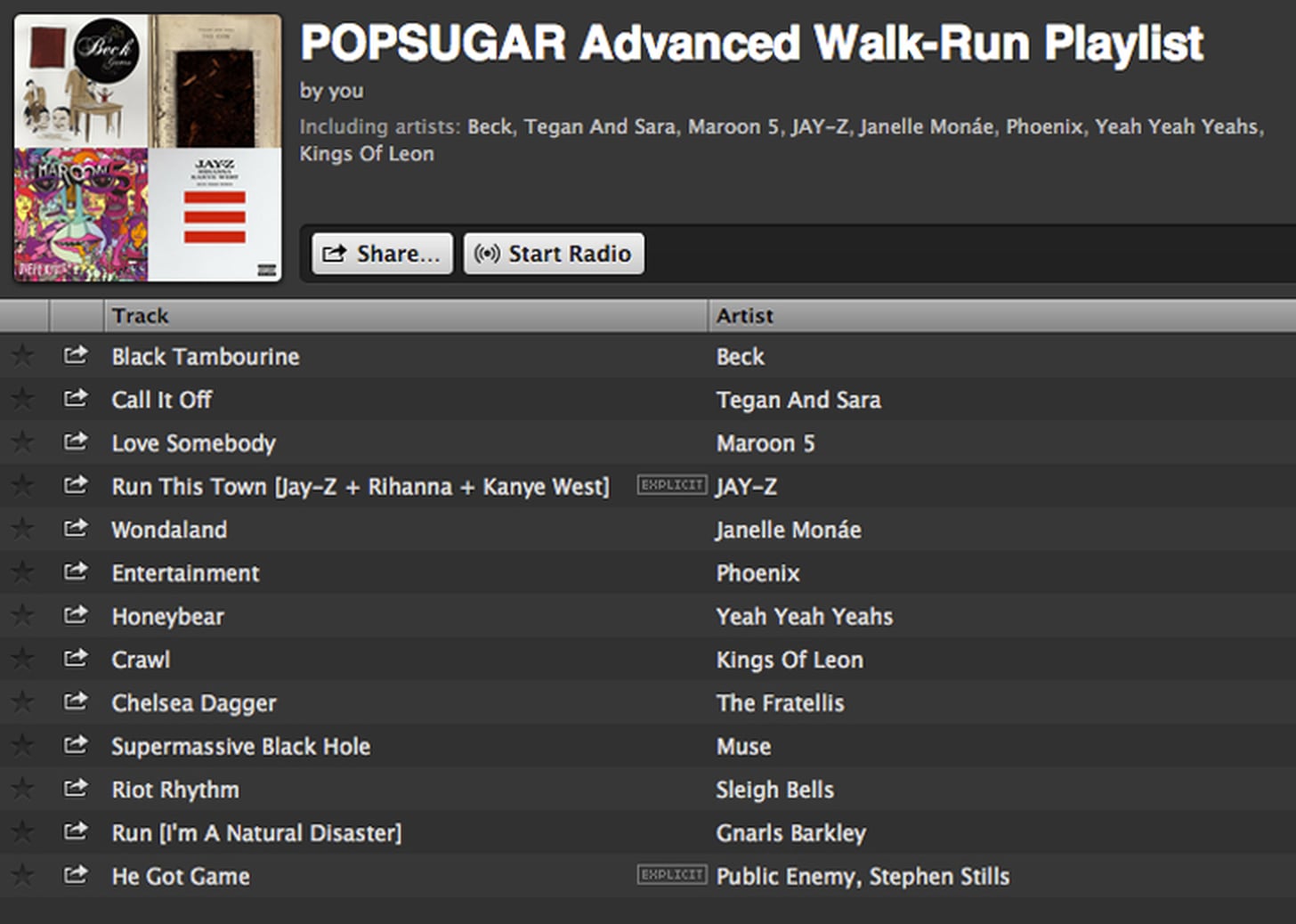Below is the cleaned-up and detailed caption for the image:

---

A screen capture from a music streaming site, possibly Spotify or Apple Music, displaying a playlist titled "Pop Sugar Advance Walk Run," curated by the user. On the left side of the image, three album covers are prominently featured. The first is Beck's album, featuring a somber scene with people gathered around a desk and a tan and brown color palette. Next, a vibrant cover art from Maroon 5, characterized by an abstract geometric face in loud, bright colors including burgundy, purple, yellow, and green. Finally, Jay-Z's album cover, featuring three red bars with black font.

Below these covers, the title "Pop Sugar Advance Walk Run Playlist by You" is displayed in white text. The listed artists include Beck, Tegan and Sara, Maroon 5, Jay-Z, Janelle Monáe, Phoenix, Yeah Yeah Yeahs, and Kings of Leon. Two white buttons with black font are visible: "Share" with a square icon featuring an arrow, and "Start Radio" with a circular icon emitting wave-like lines.

On the right side, a gray bar separates the track details. The columns are labeled "Track" and "Artist," and each track is marked with an asterisk icon and a share box icon. The playlist tracks, all listed in white font, include:

1. "Black Tambourine" by Beck
2. "Call It Off" by Tegan and Sara
3. "Love Somebody" by Maroon 5
4. "Run This Town" by Jay-Z featuring Rihanna and Kanye West (explicit)
5. "Wondaland" by Janelle Monáe
6. "Entertainment" by Phoenix
7. "Honey Bear" by Yeah Yeah Yeahs
8. "Crawl" by Kings of Leon
9. "Chelsea Dagger" by The Fratellis
10. "Supermassive Black Hole" by Muse
11. "Riot Rhythm" by Sleigh Bells
12. "Run (I'm a Natural Disaster)" by Gnarls Barkley
13. "He Got Game" by Public Enemy featuring Stephen Stills (explicit)

This detailed caption captures the visual and textual elements of the playlist screen, providing a comprehensive description of the image.